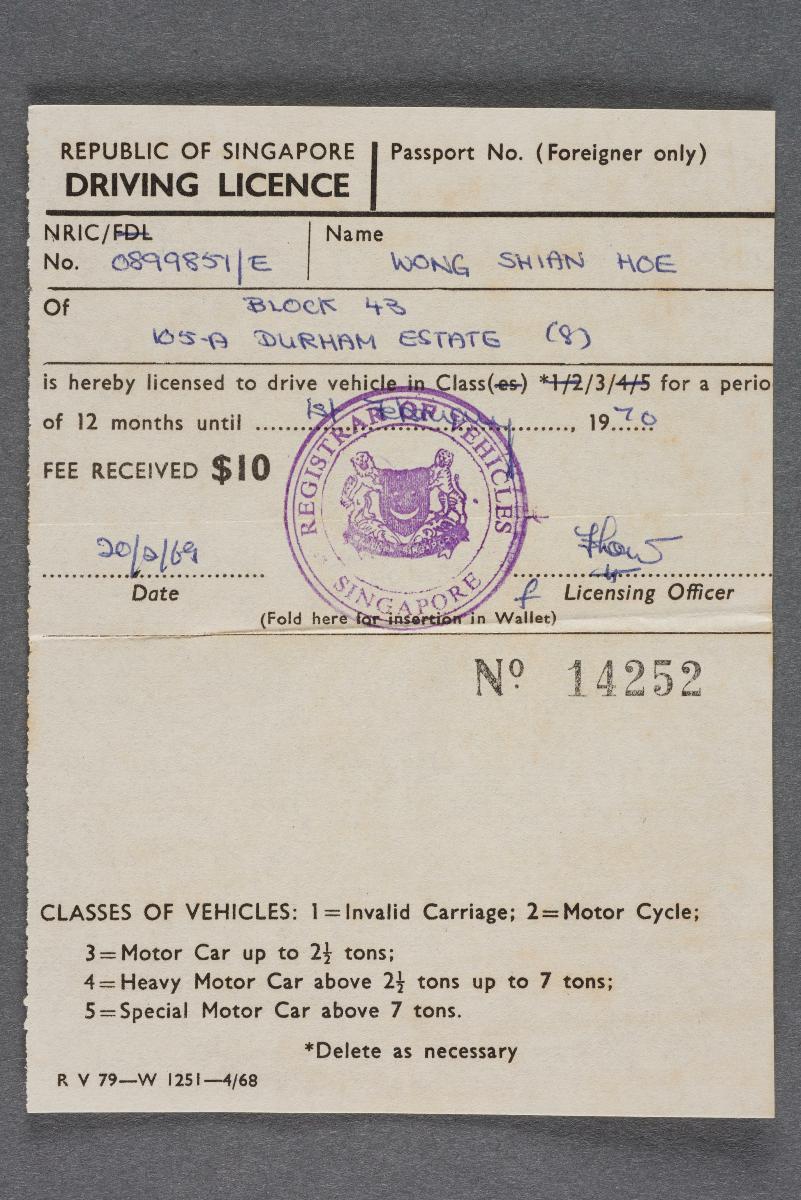The image is a photo of a Republic of Singapore driving license document. At the top left, it reads "Republic of Singapore Driving License." Below that, there is a section for "Passport Number" which is reserved for foreign applicants but is left blank in this case. The license details are filled in with blue ballpoint pen: the NRIC/FDL number is 0899851/E, and the license holder's name is Wong Hsien Ho. 

Wong Hsien Ho resides at Block 43, BSA Durham State (8). This license authorizes Wong Hsien Ho to drive vehicles in class 3, while classes 1, 2, 4, and 5 are crossed out. The license is valid for a period of 12 months until a partially obscured date in 1970, due to a stamp covering the exact day and month. 

The fee of $10 was received on the date 22/69, indicated by a stamp from the Registrar of Vehicles Singapore, along with a licensing officer's signature. The document also contains instructions "Fold here for insertion in wallet," and a stamped number 14252. 

The classes of vehicles are listed at the bottom: 1) Invalid Carriage, 2) Motorcycle, 3) Motor Car up to 2.5 tons, 4) Heavy Motor Car above 2.5 tons and up to 7 tons, and 5) Special Motor Car above 7 tons. The license includes an asterisk noting "delete as necessary" for the various vehicle classes.